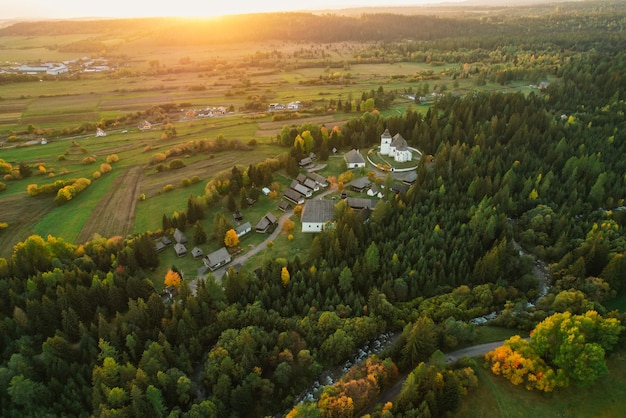This aerial photograph, likely taken from a drone or airplane, captures a vast and lush landscape transitioning into early fall. The scene stretches out into the distance towards a soft mountain range, where the amber hues of the setting sun cast a warm glow across the image. The upper portion of the photo shows bright light indicating sunset, with a light blue sky blending into an amber horizon.

Dominating the scene are expansive forests, primarily composed of dark green trees, interspersed with patches of yellow and orange foliage, hinting at the onset of autumn. Towards the bottom right corner, a curving road is visible, partially obscured by the thick canopy of trees. Nestled within this forest are clusters of gray-roofed houses, including a prominent large white house or church with a steeple, situated on a circular, elevated plateau flanked by orange-colored trees.

Beyond the dense woods, the landscape opens up to scattered fields and farmland, indicating sparse population density. The well-manicured lawns and structures suggest an affluent estate, meticulously maintained, perhaps spanning several acres. This serene, green, and beautiful scene, complemented by the glow of the setting sun, epitomizes a picturesque and pastoral setting at the verge of fall.